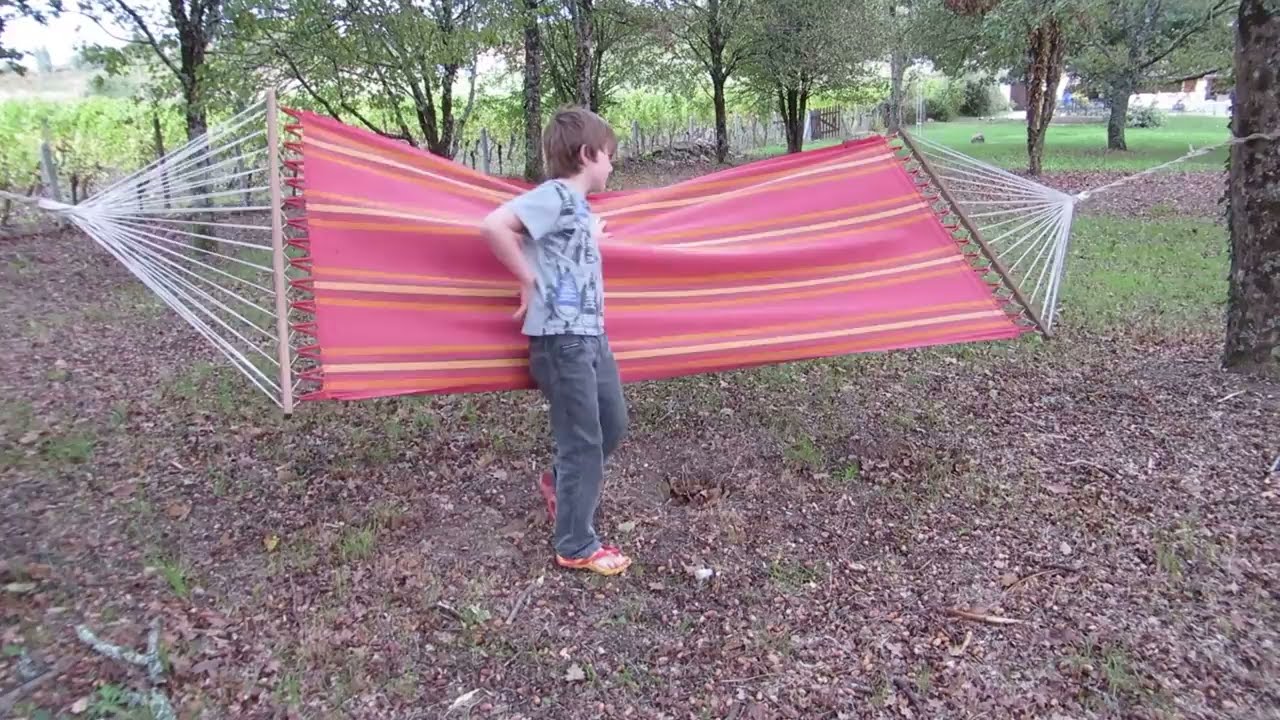This landscape-oriented photograph depicts a young boy, approximately 11-12 years old, standing in front of a vibrant hammock in what appears to be a large backyard. The boy, who has light skin and brown hair, is dressed in a light grayish T-shirt adorned with a design, black jeans, and sandals. He is shown in a side profile, facing to the right, while leaning slightly against the hammock. The hammock itself is richly colored with horizontal stripes of red, orange, pink, and yellow, and is supported by two wooden bars connected to white ropes, which are tied to trees on either side. Due to the boy's weight, the hammock is tilted upward towards the camera. The background reveals a park-like setting with numerous trees and a grassy landscape, suggesting a spacious, maybe rural environment that could also be part of a large backyard. The ground beneath the hammock consists of dirt and leaves, enhancing the natural, outdoor atmosphere of the scene.